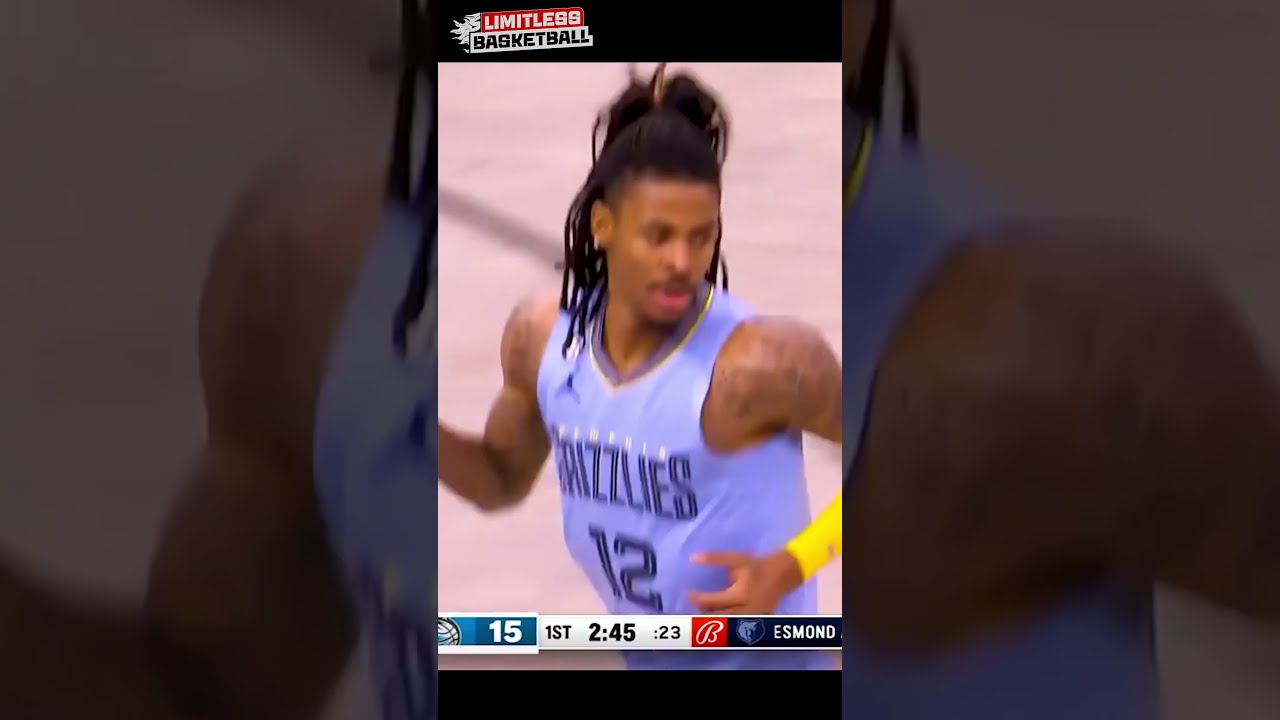The image is a blurry screenshot of a basketball game viewed on a cell phone in portrait orientation. At the top left corner, there's a logo with white and black lettering on a red and white background that reads "Limitless Basketball." The main focus of the screenshot is a black male basketball player with shoulder-length dreadlocks partially tied back, revealing a mustache, tattoos on both arms, and an earring in his right ear. The player is wearing a light blue jersey with the word "Grizzlies" and the number 12 formatted in a darker blue font. Additionally, he has a bright yellow sleeve on his left forearm. Along the bottom of the screen, a banner displays the game score: "15" followed by "First," "2:45" indicating the minutes remaining, "23" seconds, and a "B" logo next to the word "Esmond." The background faintly shows a section of the basketball court.